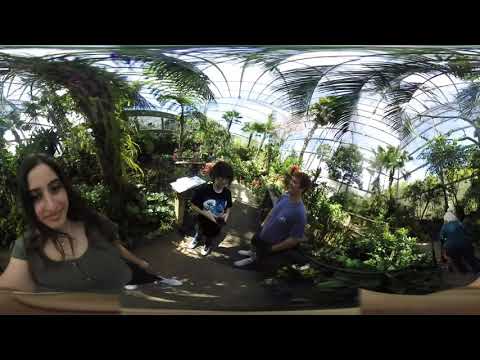In a bright, glass-domed greenhouse or botanical garden, a lively scene unfolds. On the left, a smiling woman with long, dark curly hair wears a brown button-down short-sleeved shirt. Her arm stretches out across the bottom of the frame, suggesting she might be taking the photo. In the center of the image, two people stand close together: one in a black short-sleeved shirt and the other in a blue short-sleeved shirt. The background features a pristine white structure with black lines weaving through it, almost like a steel framework. This area is teeming with lush, diverse greenery. Green leaves of varying sizes and shapes—some tall, some short—surround the individuals, extending upwards towards the domed roof. Exotic plants, possibly from tropical regions, add to the vibrant atmosphere, contrasting beautifully against the white and black background. The overall scene is slightly blurred, adding a dynamic and candid feel to the moment captured within this verdant sanctuary.